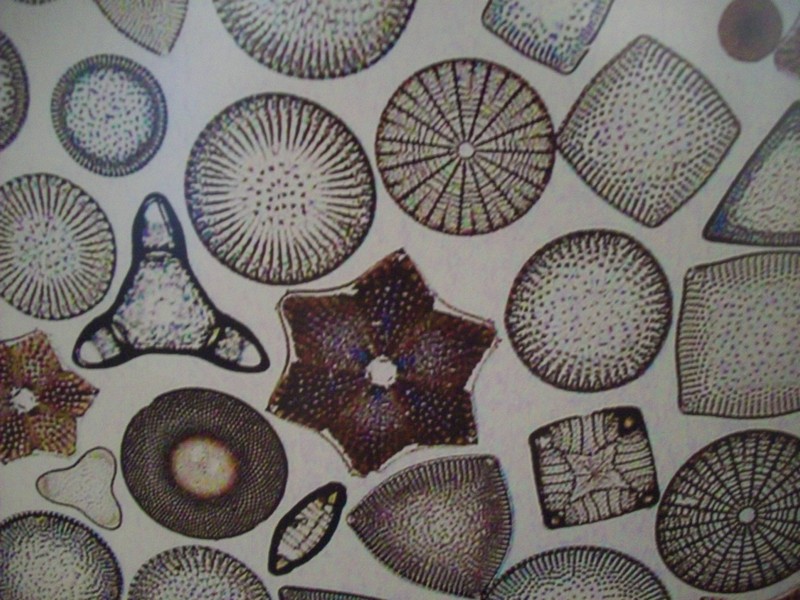The image is a detailed, hand-drawn artwork set against a white background, featuring an array of distinct and vibrant shapes. At the center of the image is a brown, six-petaled flower shape adorned with blue dots, and its center is white. Flanking this flower are black-outlined triangles embellished with green and blue dots. To the right of the flower is a circular pattern filled with numerous brown dots, while beneath the flower is an oval shape with horizontal lines resembling a football. Additionally, the drawing includes a variety of seashells and sea stars, which are intricately detailed and colored in hues of red, green, black, dark red, purple, and blue. The overall composition includes a plethora of unique shapes such as circles, hexagonal patterns, boomerang-like designs, triangles, and squares, all contributing to a rich and diverse visual tapestry.